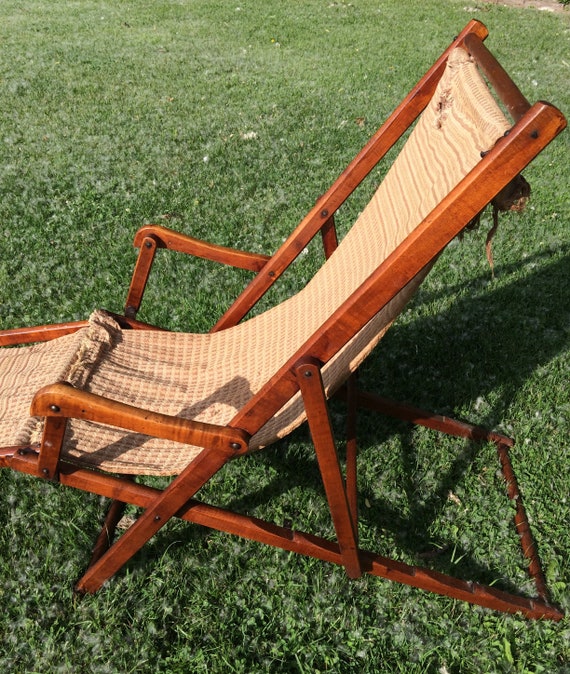This outdoor photograph showcases a homemade wooden lawn chair situated on a vibrant green grass lawn under daylight. The chair, constructed from dark brown wood, features a brown and white striped fabric that appears bunched at the leg area, giving it an unprofessional look. The fabric, not plastic, is attached to the chair, which is long and designed for lounging, though it doesn't fully fit within the frame of the picture. The grass is cut short, lush, and devoid of leaves, providing a clean and lively backdrop. The chair casts a shadow on the grass behind it, highlighting the sunny conditions, though the sky is not visible in this focused ground-level shot.